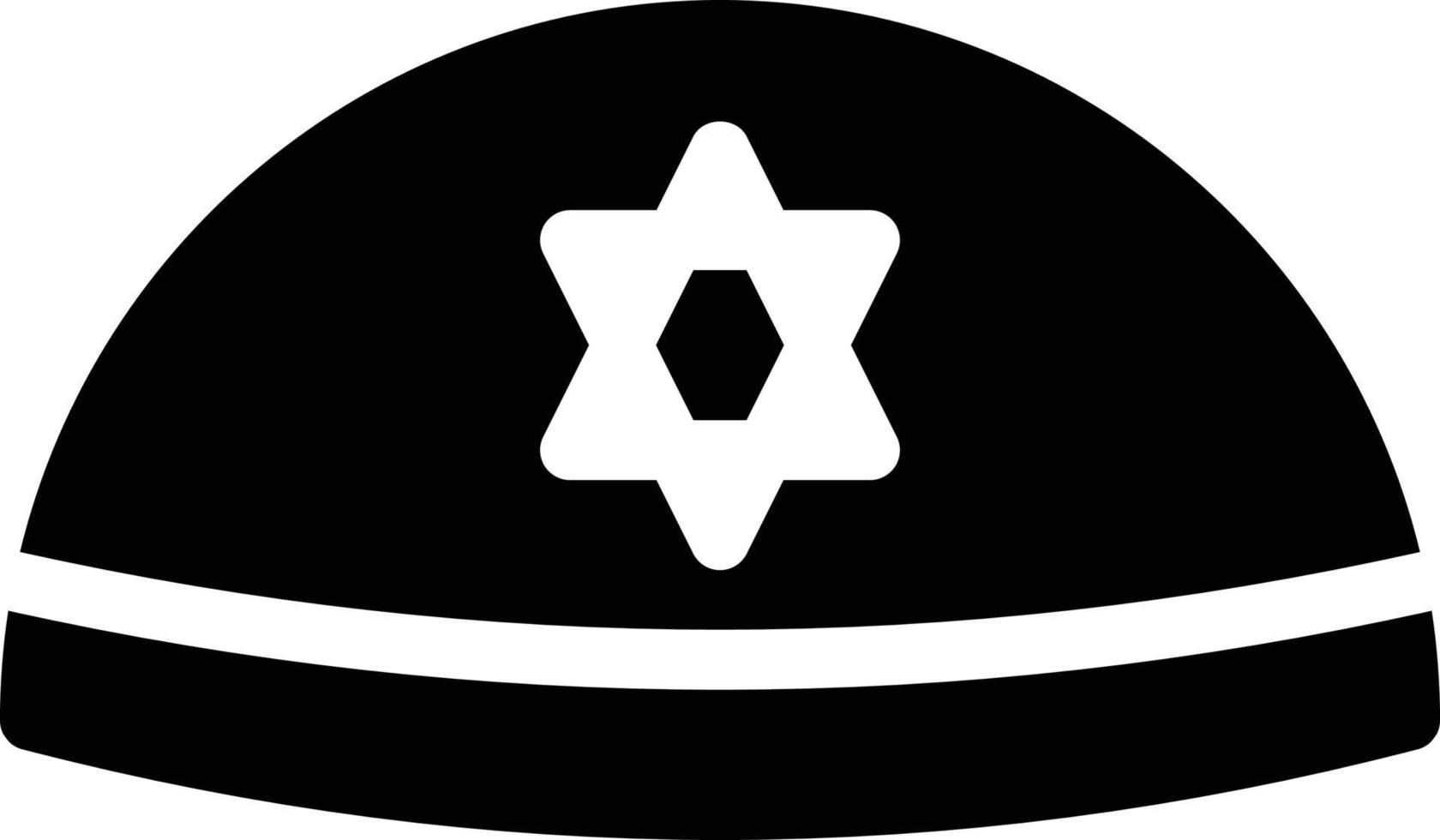The image depicts a 2D drawing of a Jewish kippah rendered in black and white. The kippah is represented as a half-circle with the rounded edge at the top and the flat edge at the bottom, giving it a slightly helmet-like appearance. The top and bottom horizontal edges of the overall rectangular image are approximately three times longer than the vertical sides. A distinct white stripe runs horizontally across the bottom portion of the kippah. Dominating the top center of the kippah is a six-pointed Star of David, which is white with a black hexagon at its center. The simple yet symbolic design is set against a completely white background.